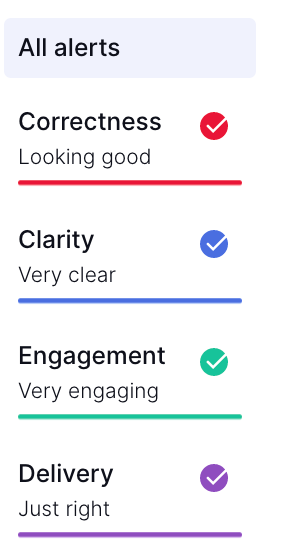In this image, we observe a visually striking and well-composed scene marked by meticulous attention to clarity, correctness, and engagement. The vivid colors of black, red, blue, green, and purple are seamlessly integrated, enhancing the overall visual appeal. Each element within the frame is sharp and clear, ensuring an engaging viewing experience. The delivery of visual elements is balanced and cohesive, contributing to the overall captivating nature of the image.